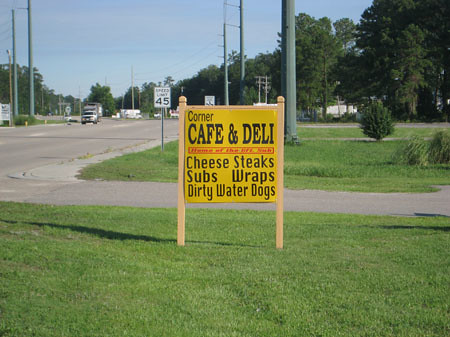A photograph captures a suburban street scene. Prominently displayed on a well-kept lawn is a sign with two tan wooden posts supporting a square yellow sign. The sign reads "Corner Cafe and Deli" in bold lettering. Below this, a red outlined box contains partially obscured red text that is difficult to decipher. Further down in black text, the sign lists various menu items: "Cheesesteaks, Subs, Wraps, Dirty Water Dogs." In the background, a speed limit sign indicating "45" is visible along with a car driving down the road. The surrounding area is typical of a suburban neighborhood, featuring paved roads and neatly trimmed grass.